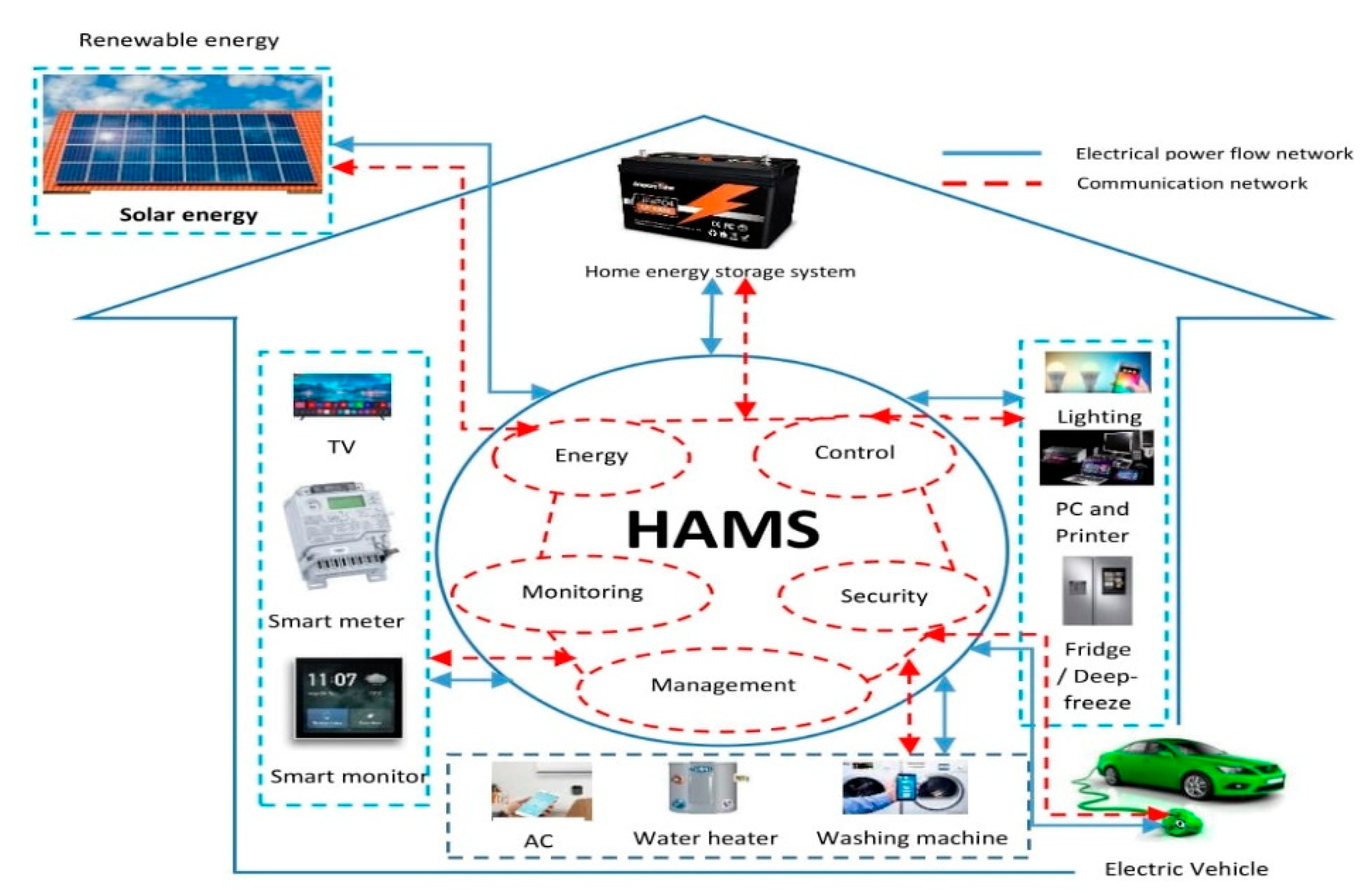This detailed diagram presents a comprehensive look at a home electricity system. At the top left, an image of solar panels symbolizes renewable energy, depicted with a dark blue hue surrounded by an orange border. These panels likely comprise four rows of eight cells each. Directly beneath the house's roof, a home battery storage system is illustrated. An array of various components, including a smart meter, TV, lighting, a freezer, and a refrigerator, are spread throughout the house's outline. This house illustration is primarily drawn with a blue outline on a white background. 

Central to the diagram is a blue circle encompassed by numerous arrows pointing in multiple directions, labeled with “energy,” “control,” “security,” “management,” and “monitoring.” These terms are circled with red dashed lines and connected to the acronym “HAMS.” Also highlighted are the dual networks within the system: a solid blue line represents the electrical power flow network while dashed red lines signify the communication network.

The bottom right corner of the diagram features an electric vehicle, showcasing its integration into the home electricity ecosystem. Various other home appliances such as an air conditioner, water heater, washing machine, PC, and printer, are also included. Overall, this visual intricately details the interplay and control mechanisms of modern home energy systems, emphasizing renewable energy sources, energy storage, and smart home management.